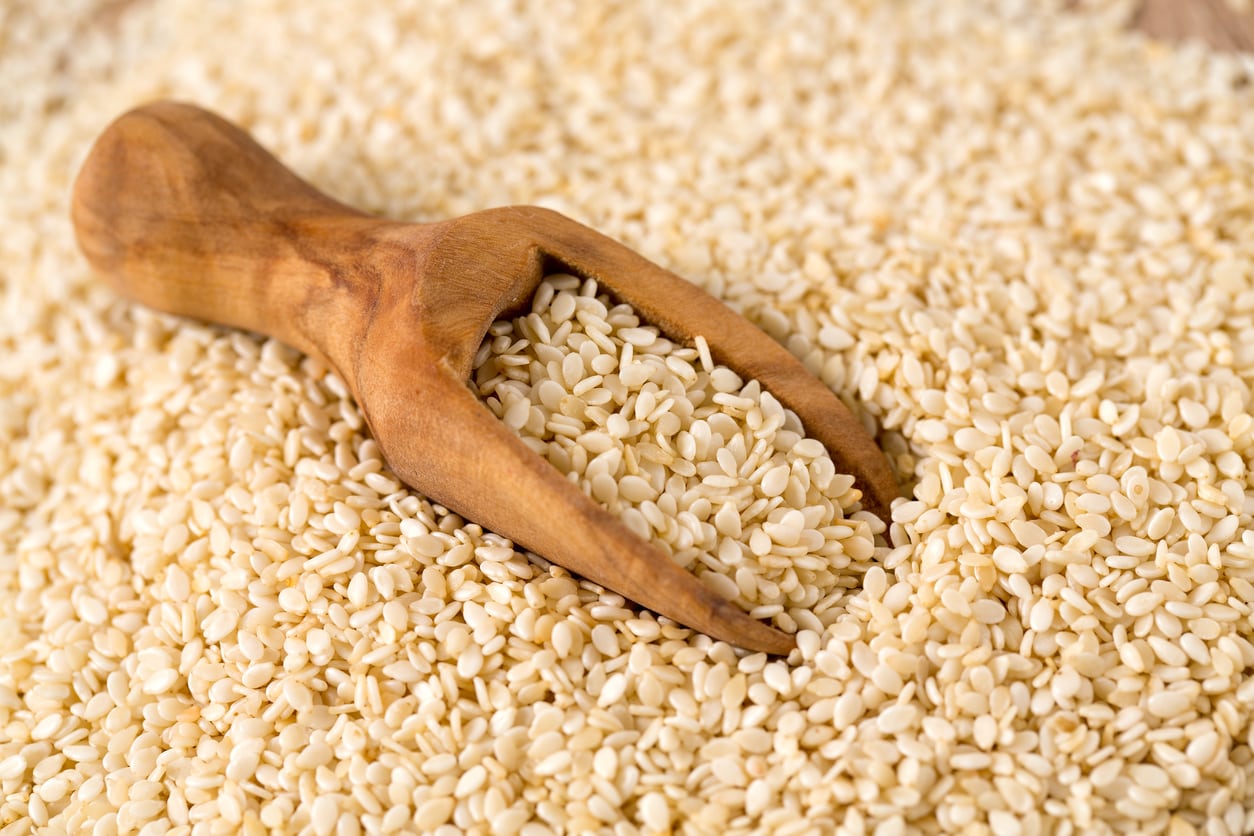The image features a detailed close-up of a pile of tiny, light beige, oval-shaped grains, slightly golden in color, covering the entire frame. Dominating the center is a hand-carved wooden scoop with a rounded handle and a rectangular scooping area, nestled within the grains. The grains could be sesame seeds, but they share characteristics with oats or a similar type of small grain, evident in their off-white hue. The grains appear sharp in the foreground, but blur slightly towards the top of the image due to depth of field. The scene is well-lit, creating a natural and appealing contrast between the wooden scoop and the grains. In the upper right corner, there is a hint of a wooden surface, though it remains indistinct and blurry. The overall setting is bright, clear, and focused solely on the grains and the scoop, evoking the idea of a rustic display or an invitation to fill up a bag using the scoop.